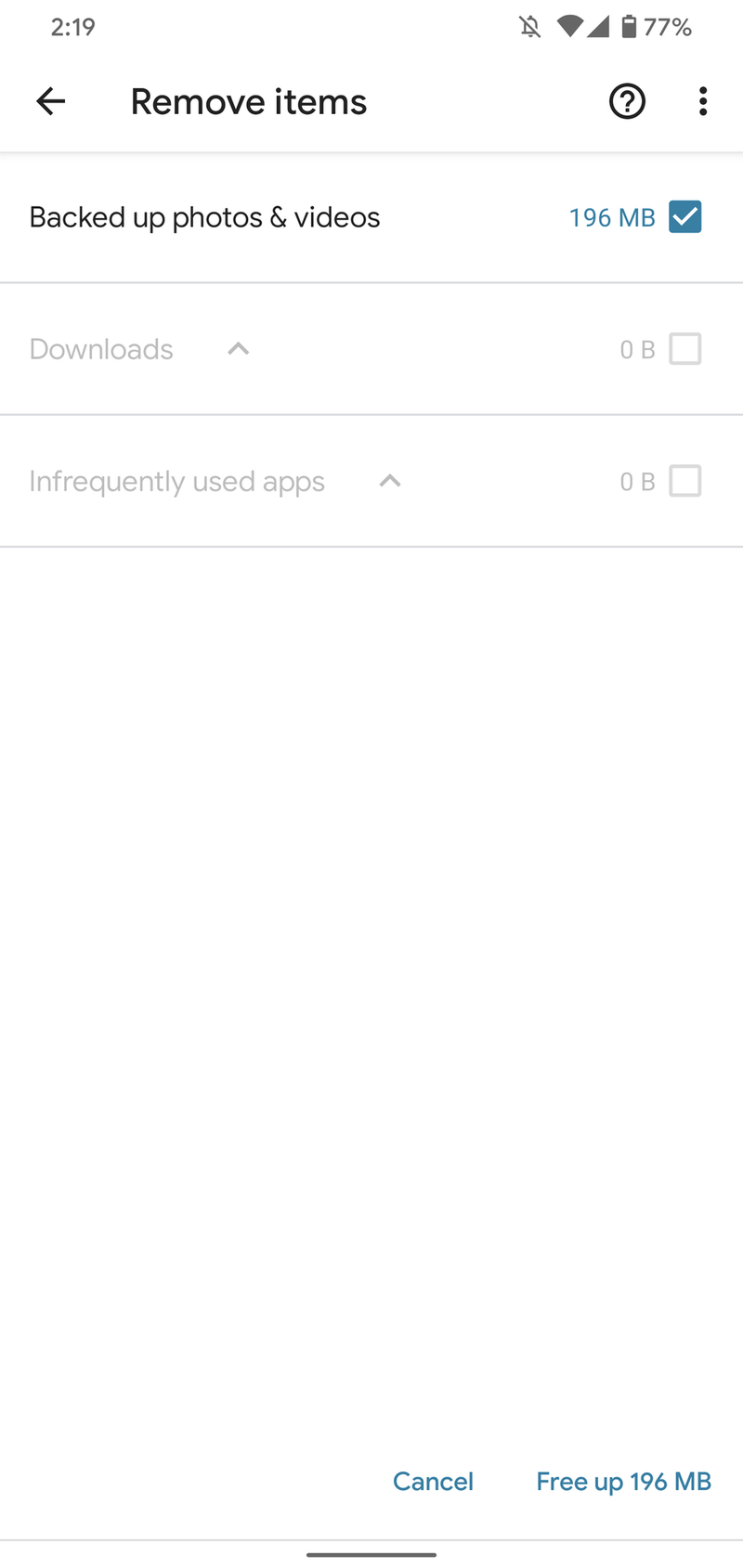The image is a screenshot taken from a smartphone, displaying a data management interface. At the top of the screen, the status bar shows the current time (2:19) alongside icons for an alert (a bell with a slash through it, indicating mute), Wi-Fi connectivity, and battery life, which is at 77%.

Below the status bar, there are various interface elements for navigating and managing data. On the top left is a left arrow for going back, followed by buttons for "Remove Items" and a circled question mark for help. To their right, there are three vertical dots indicating additional options.

The main content area is divided into three sections, though only one is active at the moment. The currently selected option is "Backed up photos and videos," marked by a white check mark within a blue box. This section displays "196 MB" in blue text, representing the data size.

The subsequent two sections are "Downloads" and "Infrequently used apps." Both are inactive and grayed out, with "Downloads" showing "0 B" and "Infrequently used apps" not displaying any data size.

The background of the interface is white, while most of the text is black, except for the text and boxes in the grayed-out sections, which are light gray. Additionally, the blue elements draw attention to the active choices and primary actions.

At the bottom of the screen are two buttons: "Cancel" on the left, which is in blue text, and "Free up 196 MB" on the right, also in blue text, guiding the user to either cancel the action or proceed with freeing up storage.